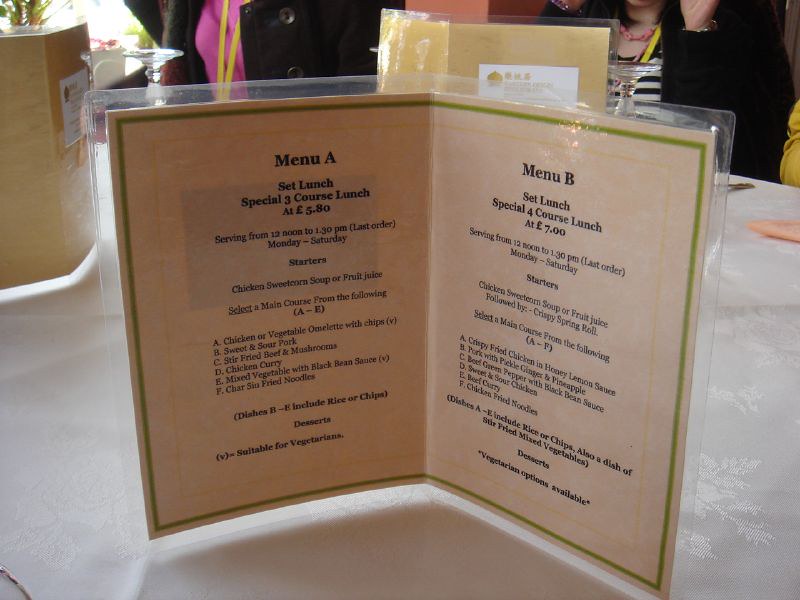This photograph captures a detailed arrangement at a restaurant table featuring a propped-up laminated menu. The menu, with a green and yellow border on a white cardboard, is prominently displayed in the center of the white table, showcasing two sets of lunch options: Menu A and Menu B. Menu A offers a three-course lunch for £5.80, listing starters such as chicken sweet corn soup or fruit juice, followed by several main courses labeled A to E. Menu B, set at £7.00, includes a four-course lunch with the same soup or juice starter, and additionally a crispy spring roll, offering main courses labeled A to F. Both menus indicate serving times from noon to 1:30 p.m., Monday to Saturday. 

In the background, part of a similar menu is visible, held by a person wearing a pink shirt, a yellow lanyard, and a black coat. Another individual in a white and black striped shirt can be seen, along with another menu on the far left side of the image. The setting suggests an upscale dining environment, with the clothing of the individuals and the neatly arranged tables hinting at a stylish restaurant atmosphere.